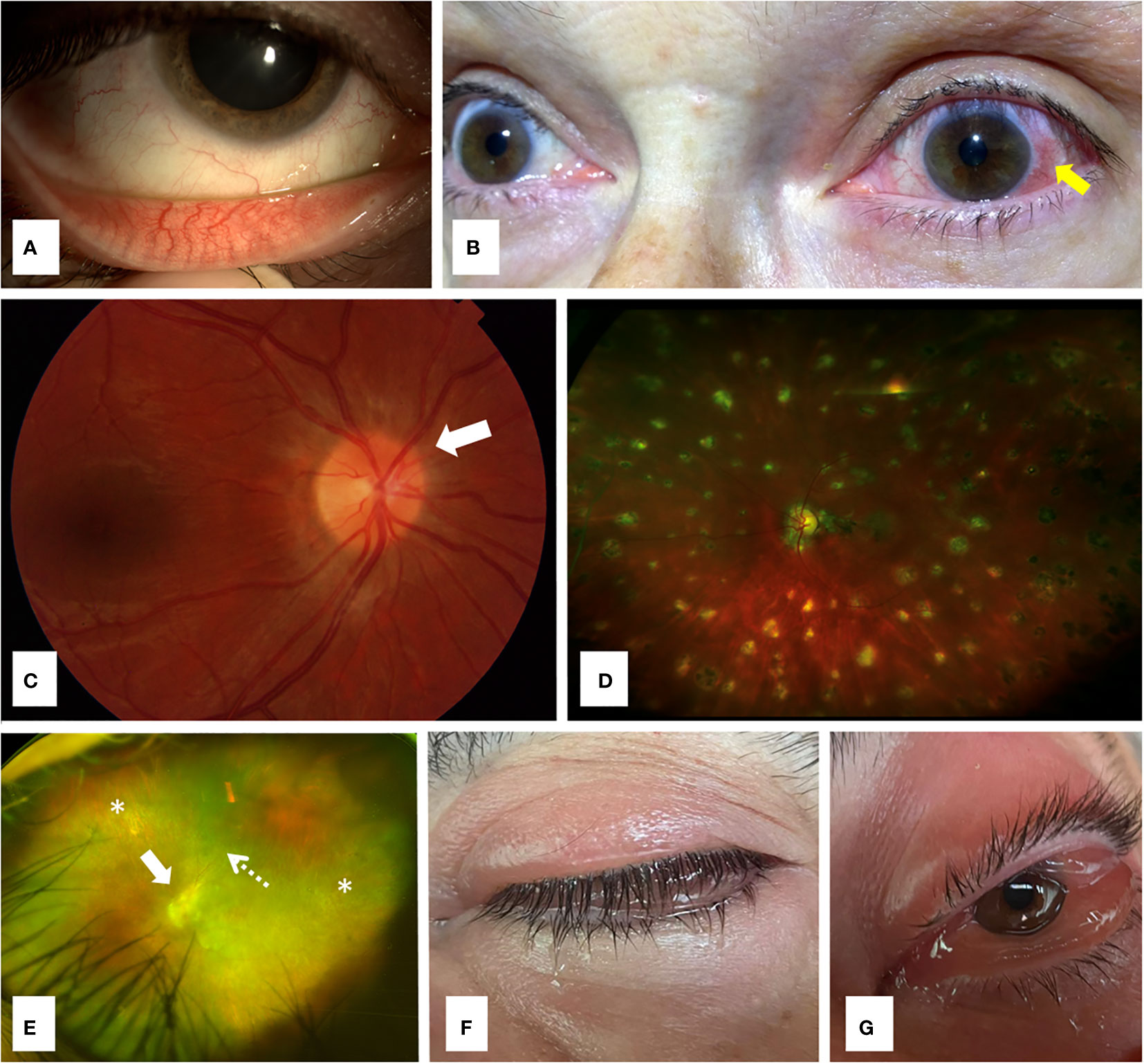The image showcases a collection of seven close-up photographs of human eyes, each labeled from A to G with a white cube bearing a black letter. 

- **Panel A:** A close-up of a green eye looking upward, with a finger pulling down the lower eyelid to reveal a light pink inner surface marred by red lines.
- **Panel B:** Both eyes of an individual, focusing on the cloudy and bloodshot left eye, highlighted by a small yellow arrow pointing to a red-lined area.
- **Panel C:** A detailed view inside an eyeball, illuminating the iris along with red lines, accented by a white arrow pointing at the illuminated section.
- **Panel D:** An extreme magnification of the eyeball, glowing orange with bright green specks throughout.
- **Panel E:** A colorful, almost fantastical section of the eye reminiscent of space, characterized by bright green illumination and multiple arrows pointing at different features, including an asterisk.
- **Panel F:** A closed eye with visible black eyelashes, tears apparent around the eyelid edges.
- **Panel G:** An eye that is fully open, yet entirely pink and gelatinous, lacking the typical white sclera.

Each photograph provides a detailed view highlighting different aspects and conditions of human eyes, from normal anatomy to various anomalies.